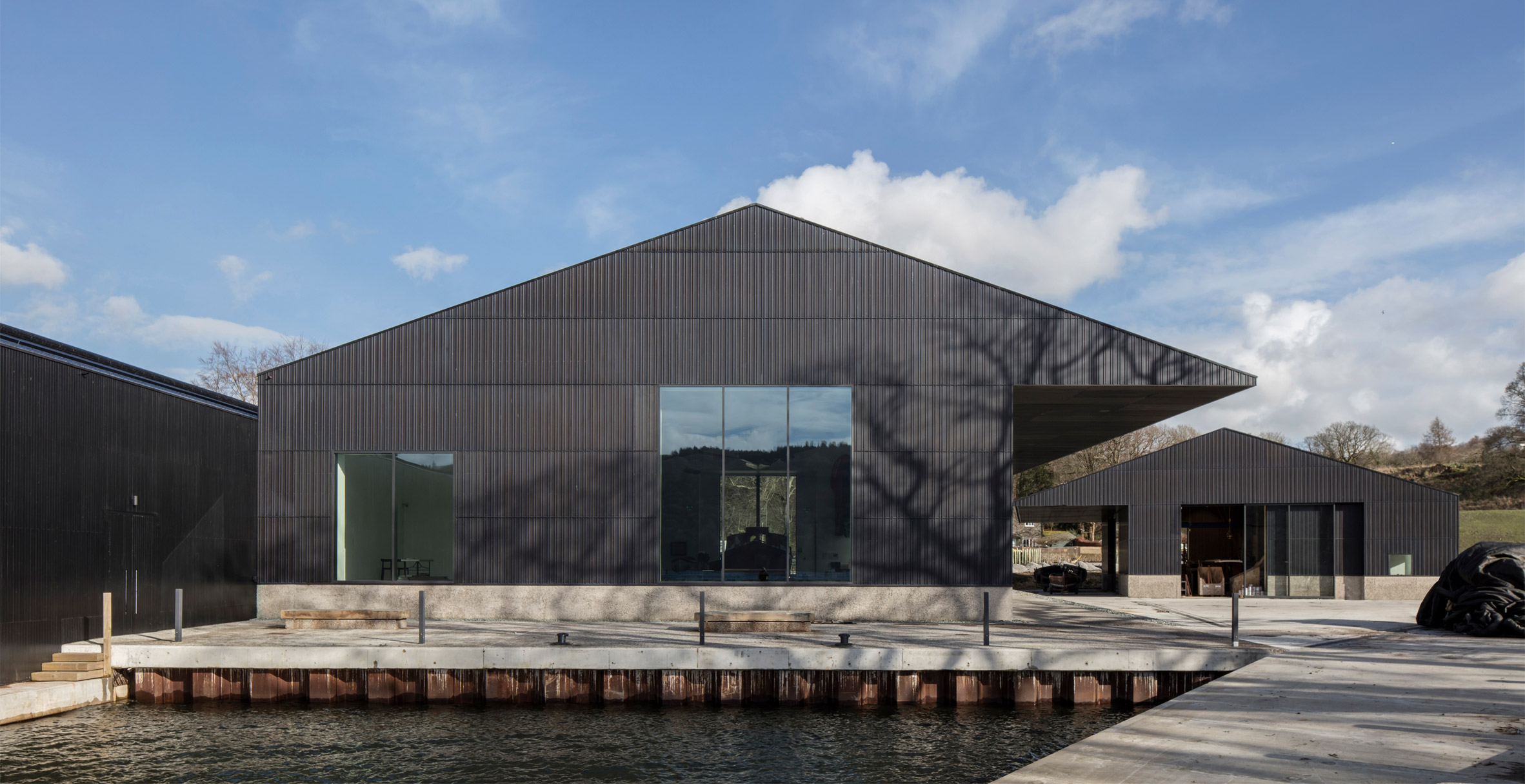The image captures a modern, industrial-style building located at a shoreline, possibly serving as a storage facility or shed for small boats. The building, constructed from gray metal, stands on a concrete surface and features a unique design with a square base and a triangular roof. Its right side is notably cut out, giving it a distinctive asymmetrical appearance. Large glass windows and a partially transparent door accentuate its modern aesthetic. In the foreground, a wooden dock extends out over a body of water, situated at the bottom left corner of the image. The scene is set during the daytime, with a light blue sky dotted with white clouds. Behind the building, grassy fields and small trees add a touch of nature to the industrial landscape.